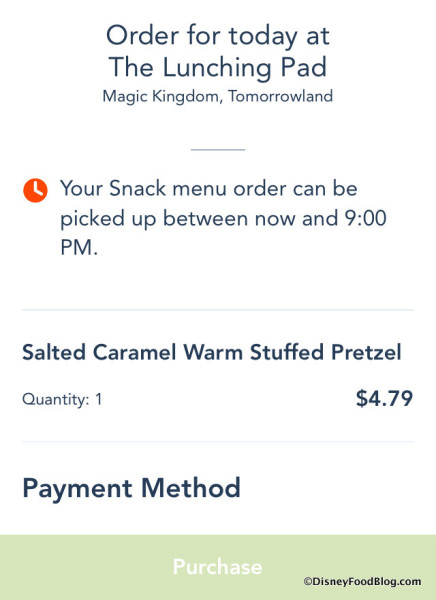A screenshot of a snack menu order from the Magic Kingdom in Tomorrowland. The top of the image features a white background with the text, "Order for lunch today at the Lunching Pad at Magic Kingdom, Tomorrowland." Below this text, a small horizontal line separates the sections. An icon of a red clock appears in the center, with the adjacent text stating, "Your snack menu order can be picked up between now and 9 PM."

Further down, a white space precedes a gray horizontal line. Below this, the order details are displayed, listing a "Salted Caramel Warm Stuffed Pretzel" with a quantity of one. To the right, the price is shown as $4.79. Underneath this item description, a heading titled "Payment Method" appears, followed by another white space.

At the very bottom of the screenshot, a light green border frames the section, with the word "Purchase" written in white centered within the border. In the bottom right corner, a small circular icon with the letter "C" is displayed next to the URL "DisneyFoodBlog.com." This screenshot details a snack menu order from a visit to the Magic Kingdom in Tomorrowland.